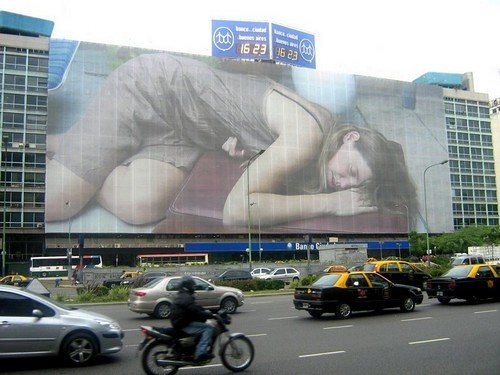This photograph captures a bustling city scene with a tall apartment or office building featuring a prominent billboard in its center. The sky above is overcast. Dominating the scene, the billboard displays a black-and-white image of a woman in a gray dress with thin straps. She is reclining on a red cushion with her legs tucked behind her and one arm beneath her head, exuding a sense of repose or melancholy. Above the billboard, a blue sign with a circle depicting stick figures and the time 16:23 in bold digits is visible. Below the building, the street is alive with activity, consisting of at least four lanes crowded with vehicles. Notably, several black taxis with yellow tops stand out, along with a man riding a black motorcycle. The vibrancy and motion of the street scene contrast with the serene yet somber depiction on the billboard, creating a compelling urban tableau.